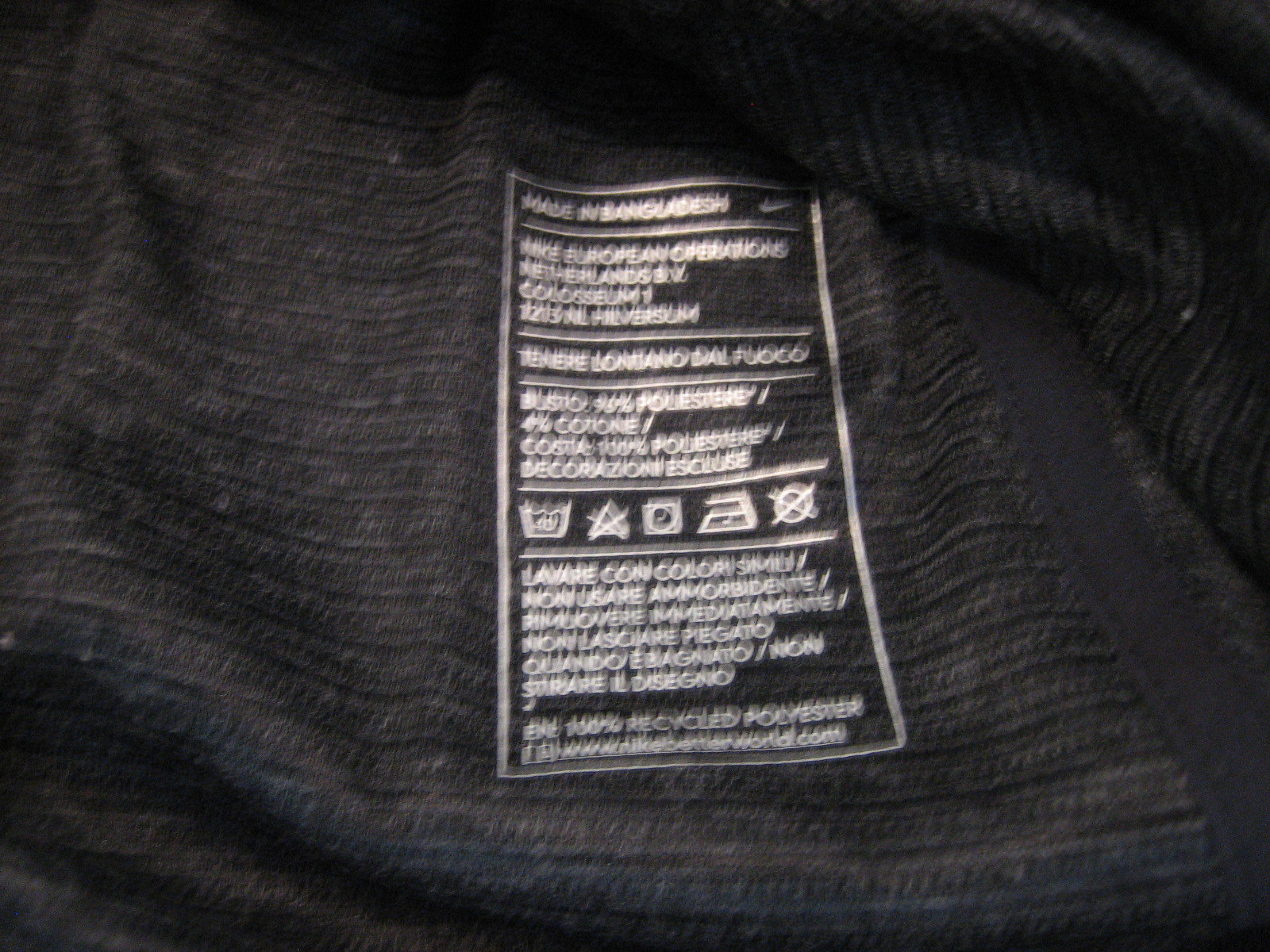This highly zoomed-in photograph showcases a black fabric item, likely a shirt, revealing detailed threads and texture indicative of a high thread count. Prominently featured is a long, rectangular tag running vertically from top to bottom. The tag is filled with white text, but the image's blur makes the writing indistinguishable. Despite the lack of clarity, the faint outline of what appears to be a Nike logo can be discerned. Alongside the text, the tag displays several icons: a basket, a star, a square with an indistinct image, an unclear icon, and a circle with an X through it. The level of zoom emphasizes the material's woven structure and the intricate details of the labeling.